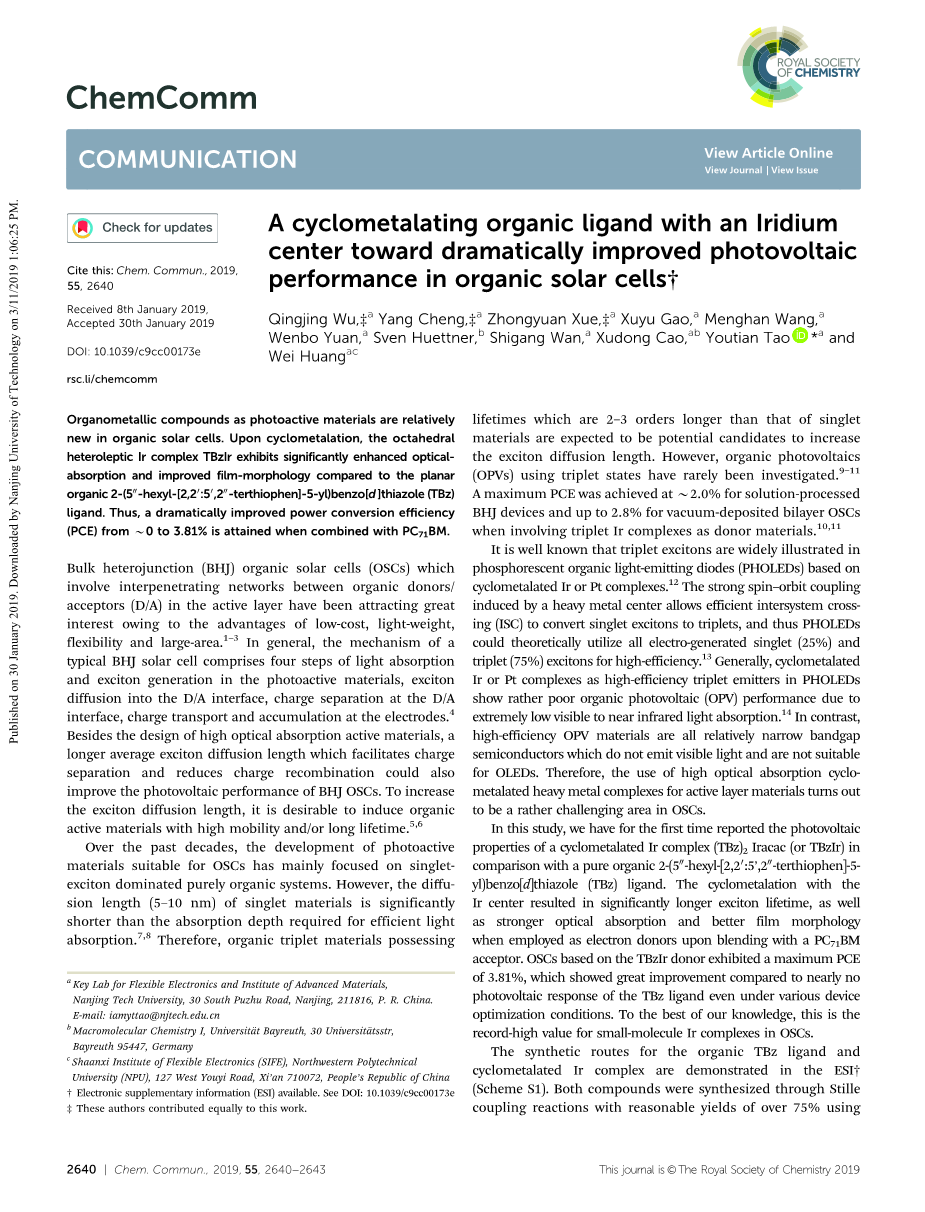The image features a detailed academic article approximately four paragraphs in length. At the top, the document is labeled "Chem Com," with "Communication" noted underneath. The title of the paper is prominently displayed, highlighting its focus on "Cyclometalline Organic Liquid with an Iridium Center Towards Dramatically Improving Photovoltaic Performance in Organic Solar Cells." The sidebar advises readers to check for updates. Citations included in the document reference "Chem Com 2019 552640" and date stamps indicating the paper was received on January 8th, 2019, and accepted on January 30th, 2019. The article delves deeper into the topic of enhancing organic solar cells with the specialized liquid, expanding on the summarized title's premise.